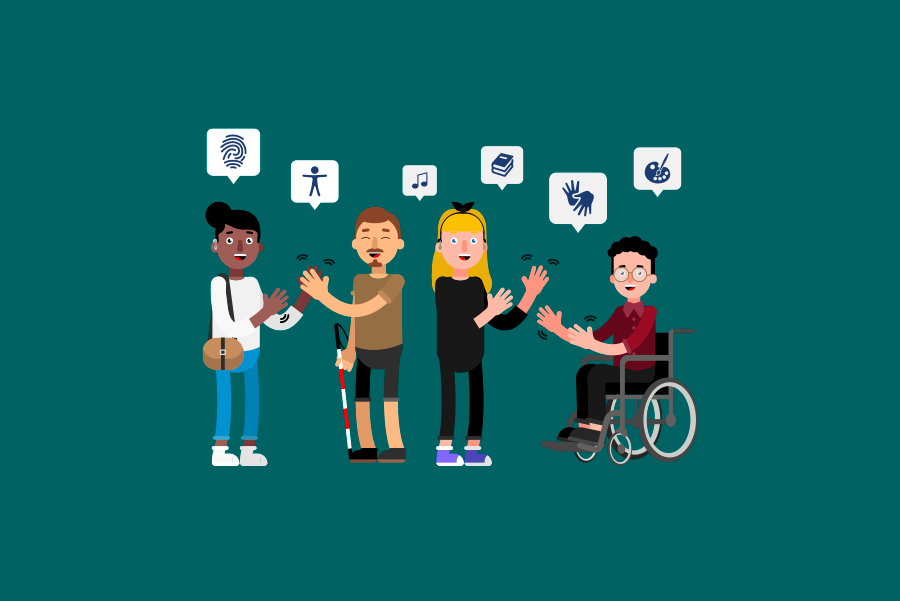The image is a computer-generated cartoon featuring four animated characters, set against a dark green background. From left to right, the characters are a woman, a man, another woman, and a man in a wheelchair. 

The first woman on the left is dressed in a white shirt, blue jeans, and white shoes, with her shoes pointing to the right while her body faces forward. She is giving a high-five with her left hand to the man next to her. This man, who appears to be blind, has his eyes closed and is holding a cane at his side. He wears a brown shirt and grey pants.

Next to him is a woman with blonde hair, clad in a black outfit with blue shoes. She appears to be clapping, suggested by marks near her hands. Finally, the man in the wheelchair is attired in a red shirt and black pants. He is facing the blonde-haired woman.

Above their heads are icons representing a fingerprint, a person, a musical note, books, clapping hands, and an easel with a paintbrush, indicating a discussion of their interests or activities. The overall style of the image is reminiscent of MS Paint or a simple computerized cartoon.